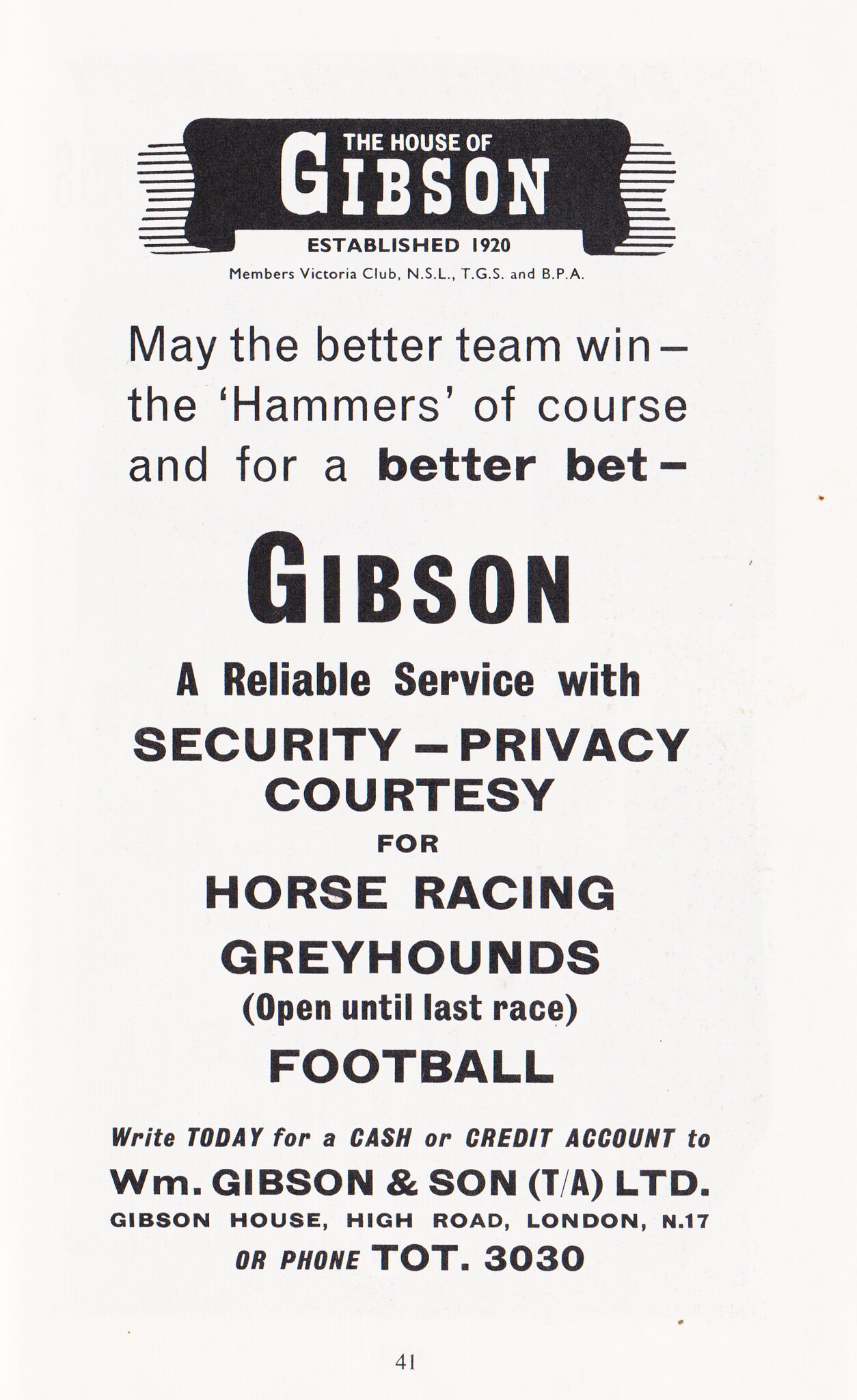The image depicts a black and white advertisement or brochure featuring a prominent heading in a black box: "The House of Gibson." Below this, it states "Established 1920" and lists memberships in the Victoria Club, NSL, TGS, and BPA. The main body of the text reads, "May the better team win, the Hammers of course, and for a better bet, Gibson." It continues with bold text proclaiming, "A reliable service with security, privacy, and courtesy for horse racing and greyhounds (open until the last race) as well as football." The contact information at the bottom instructs to "Write today for a cash or credit account to W.M. Gibson & Son, T.A.L.T.D., Gibson House, High Road, London, N17, or phone TOT 3030." The number 41 appears at the very bottom center of the page.